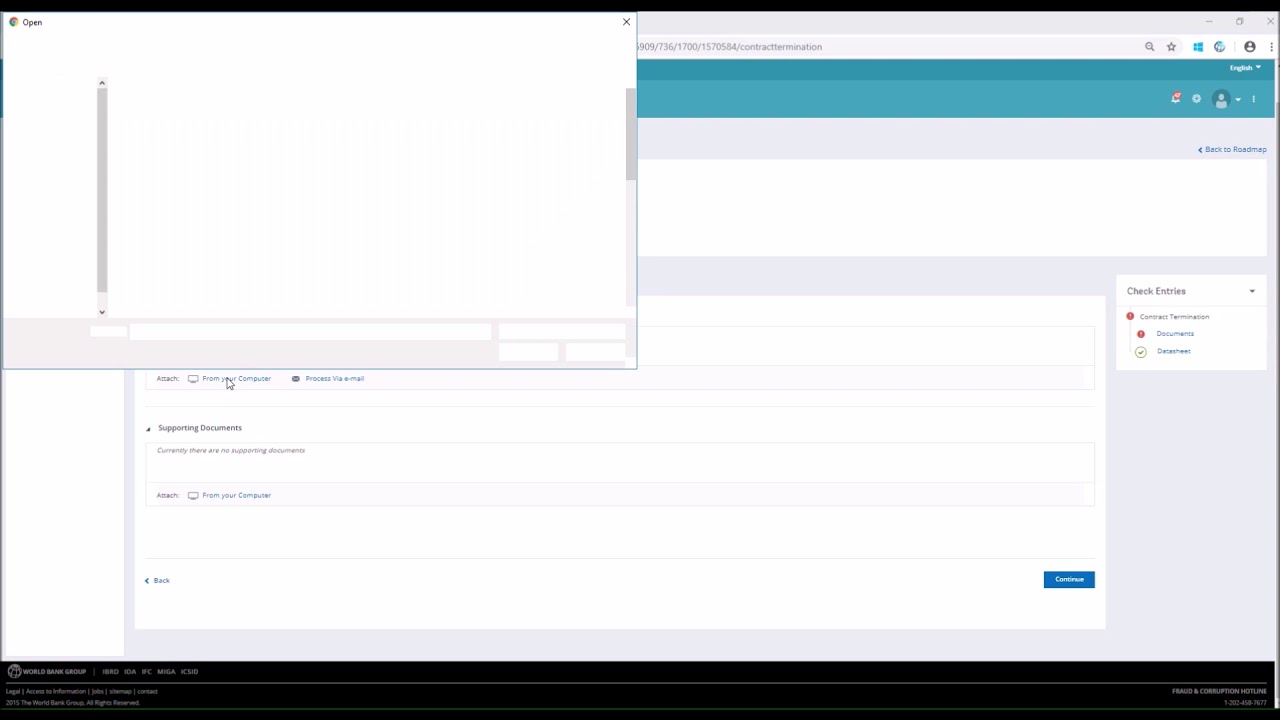Detailed Caption: 

This image depicts a partially loaded webpage featuring a variety of distinct interface elements. At the top, a broad turquoise bar stretches across the screen, though part of it is obscured by a prominent, smaller white window in the upper left corner. This obstructive window is framed with a subtle blue and gray outline and features vertical scroll bars on both its left and right sides. In the top right corner of this small white window, an 'X' button is visible, suggesting an option to close it. However, the content within the window has not yet loaded.

The main screen behind this small window appears to be the user's browsing environment, partially displaying a web address hinting at "contract termination" alongside a sequence of numbers. Adjacent to the address bar are several icons: a search icon, a star for bookmarks, a Windows icon, a globe indicating internet connectivity, and a user profile icon.

Moving downwards, more turquoise-colored icons are neatly arranged, presumably for navigation or actions such as notifications, settings, and account management. Additionally, three stars signify a menu for further options. Below these icons, a blue link prompts users to go "back to roadmap."

At the core of the page is a white box labeled with several options including "check entries," "contract termination," "documents," and "data sheet." Further below, a larger white space states that there are no supporting documents available at present. This section includes instructions for users to upload from their computer or process documents via email.

Notably, the bottom area of the screen features a blue "back" button and a more prominent blue "continue" button in the bottom right corner. Overall, the page appears incomplete, with minimal content fully loaded.